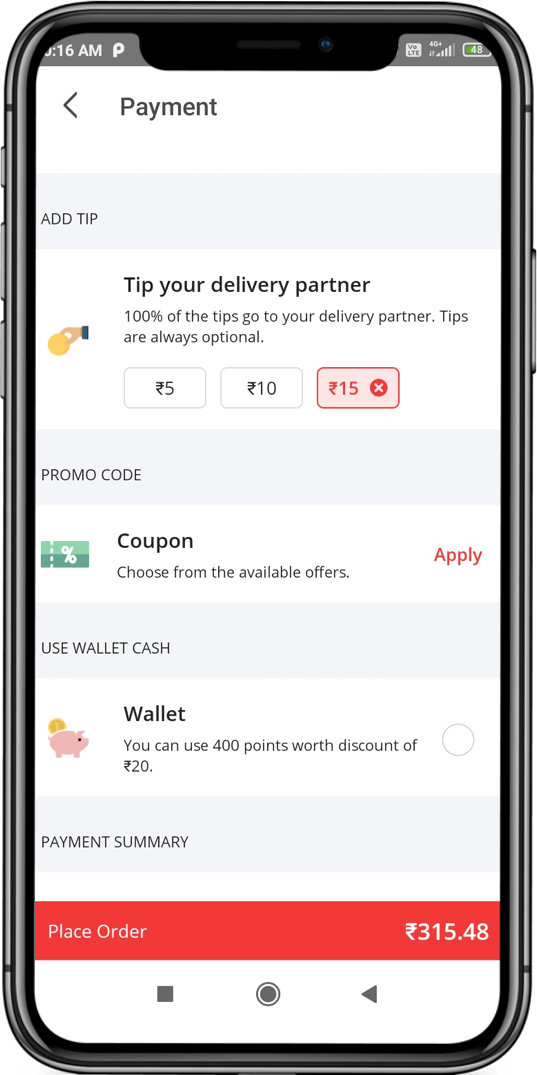Here's a cleaned-up and detailed caption for the image described:

---

The screenshot, captured at 8:16 a.m. on a smartphone, displays a payment interface. At the top, the word "Payment" is prominently featured, followed by a gray box labeled "Add Tip." Below the box, there is a message that reads, "Tip your delivery partner. 100% of the tips go to your delivery partner. Tips are always optional." Accompanying this message is a yellow hand-drawn image of a hand holding a coin.

The interface offers three tipping options in the form of buttons: £5, £10, and £15. The user has selected the £15 button. Beneath the tipping section, another gray box invites the user to enter a "Promo Code," with additional text explaining, "Choose from the available offers." The user has successfully applied a coupon, as indicated by the red text "Apply."

Following this, another gray box contains an option to "Use Wallet Cash." This section features an illustration of a piggy bank with a coin being inserted, symbolizing wallet funds. It states, "Wallet: You can use 400 points worth a discount of £20."

At the bottom of the screen, the payment summary is displayed in a gray box, followed by an orange box with the final button that reads "Place Order - £315.48." 

---

This caption provides a clear and comprehensive description of the elements visible in the screenshot.